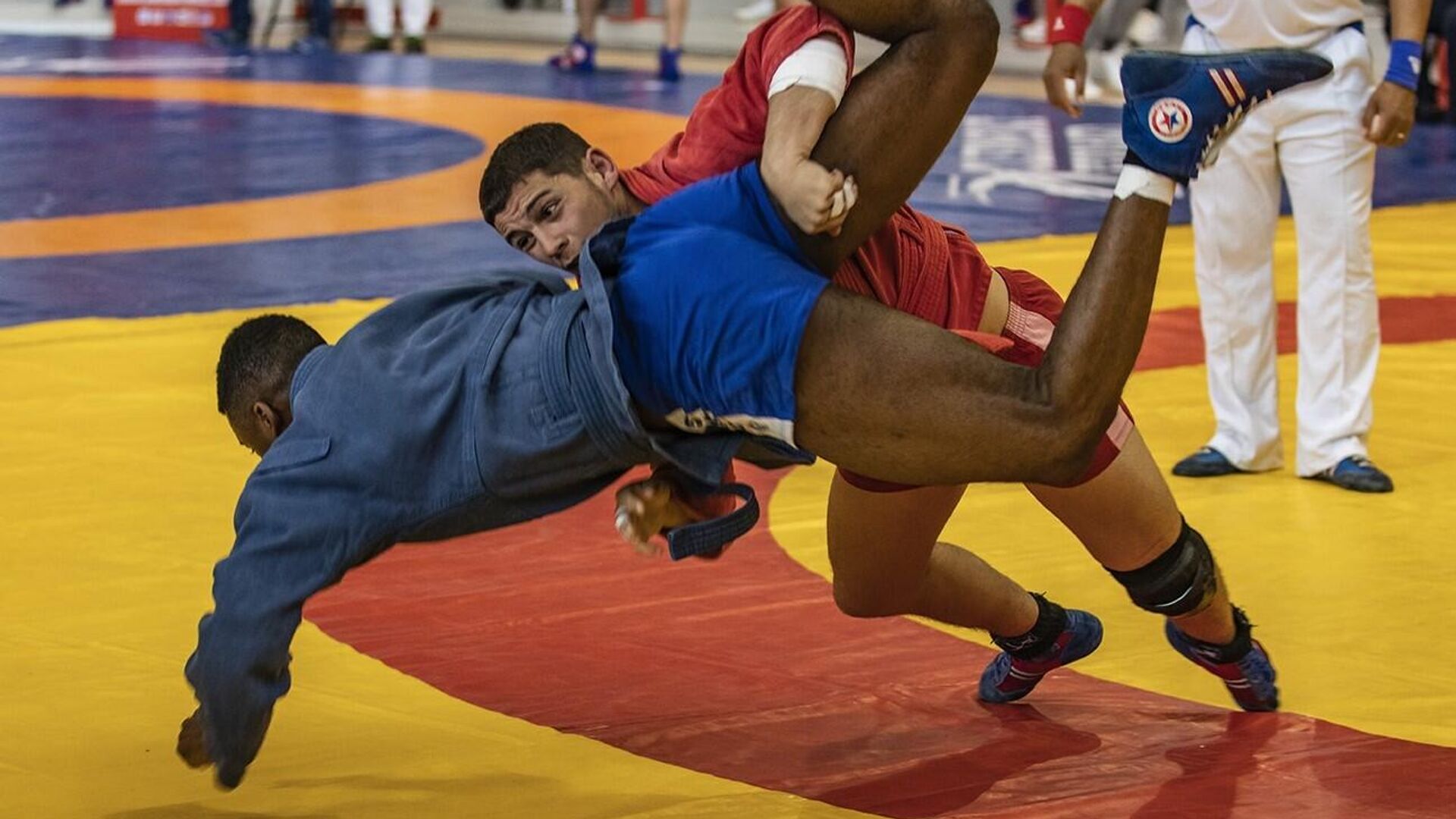In this horizontal photograph, two wrestlers are competing on a multicolored mat primarily featuring sections of red, yellow, orange, and blue. One wrestler, a black male dressed in a blue long-sleeved jacket, blue shorts, and blue high-top sneakers, is being lifted and thrown by his opponent. The opponent, a Latino male, is wearing a red long-sleeved jacket and red shorts with blue sneakers. The action takes place on a predominantly red and yellow section of the mat, with additional orange and blue areas visible in the background. A referee, clad in white pants and a white shirt, stands nearby observing the match. While spectators' feet can be glimpsed in the background, the identities of the onlookers are partially obscured due to the framing of the image. The energetic scene is captured from left to right, emphasizing the dynamic movement of the wrestlers.